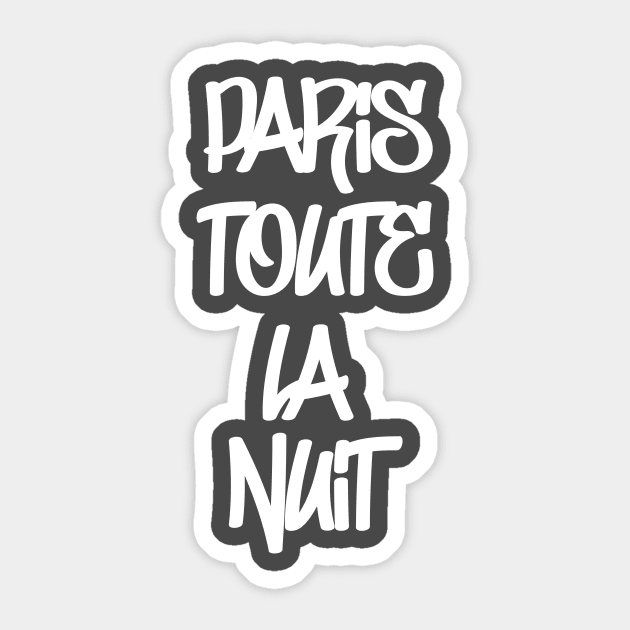The image features a bold, graffiti-style decal set against a light gray background. The striking design prominently displays the words "Paris Toute La Nuit" arranged in four stacked lines. "Paris" is at the top, followed directly by "Toute," then "La," and finally "Nuit" at the bottom. Each word is crafted in all-capital, bubble-like white letters outlined in white, with a black background within the borders of the letters themselves. This gives the text a distinctly bold and eye-catching appearance, further emphasized by the uniform sans-serif font and the centered arrangement of the words. The decal's unique shape and artistic style make it stand out, symbolizing perhaps the vibrant night life of Paris.